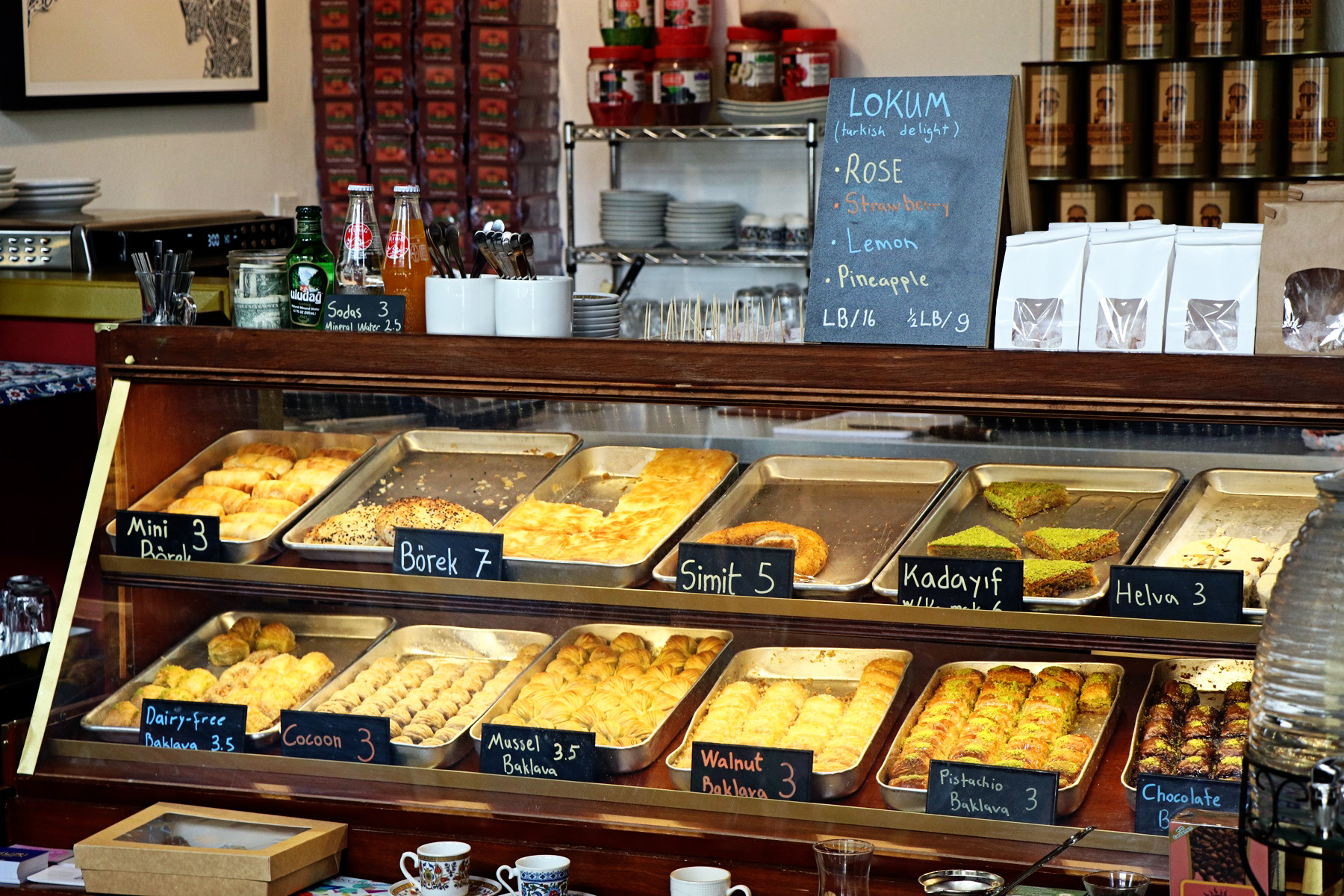The photograph captures a vibrant bakery display. Prominently featured are two glass-fronted shelves stocked with an array of pastries, each labeled with names in both English and a foreign language. Among the recognizable items are walnut baklava, pistachio baklava, chocolate baklava, dairy-free baklava, mussel baklava, and several other delicacies. Atop the display case, a chalkboard sign lists flavors of Lokum, also known as Turkish delight, with options like rose, strawberry, lemon, and pineapple, priced at $16 per pound and $9 per half-pound. The counter is adorned with white vases holding silverware, various plates, and a couple of soda bottles, identified as orange soda and green tonic. Additionally, there are small items such as toothpicks and bagged doughnuts. In the background, silver shelves hold an assortment of dishes and canisters, some of which are black and beige. The scene includes a wooden table in front of the display case, upon which small coffee cups with intricate designs are arranged next to pastry boxes. Despite the bustling setup, no staff members are visible in the photograph.